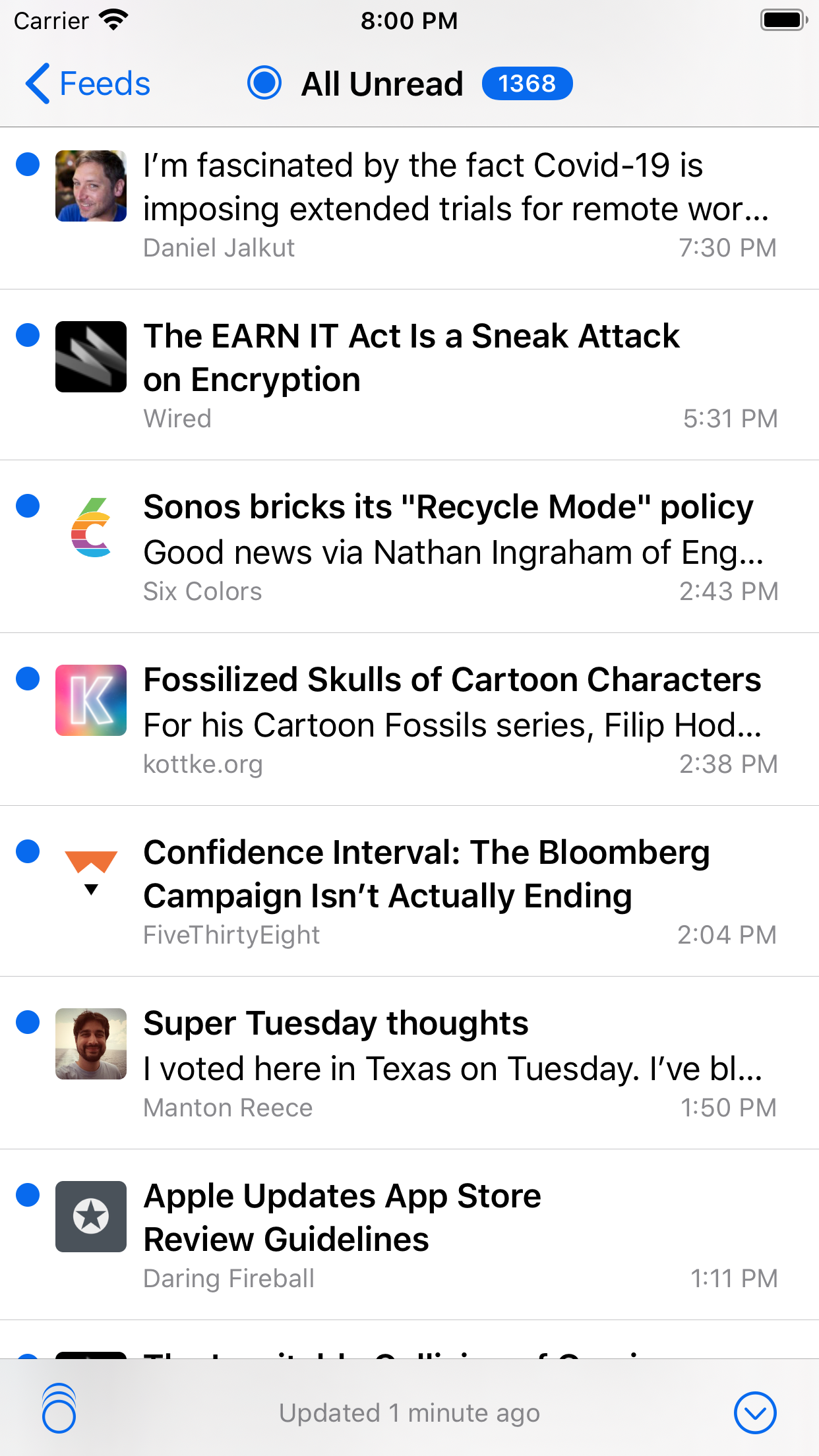This image appears to be a screenshot designed to resemble a mobile phone interface. At the top, a grey bar features the text "Carrier" in black font, suggesting a simulated phone environment. The grey bar also displays a full WiFi signal icon, the time "8:00 PM," and a full battery symbol.

Underneath the grey bar, a navigation bar appears with the word "Feeds" in blue font and a small blue arrow pointing to the left. Adjacent to this is a blue circle with the text "All" in black font set against a red background. Next to it, a blue oval containing the number "1368" in white font indicates the number of entries or notifications.

The screenshot lists several entries in a feed format. The first entry, posted at 7:30 PM, notes, "I'm fascinated by the fact COVID-19 is imposing extended trials for remote work," authored by Daniel Jalkut. To the left of this entry is a small square displaying an image of a white man with a smiling face.

The second entry, timestamped at 5:31 PM, reads, "The EARN IT Act is a sneak attack on encryption," sourced from WIRED.

The third entry reports, "Sonos bricks its recycle mode policy, good news," via Nathan Ingram of ENG, posted by 6colors at 2:43 PM.

This elaborate feed provides detailed timestamps and authors, conveying current discussions and news topics in a structured format.